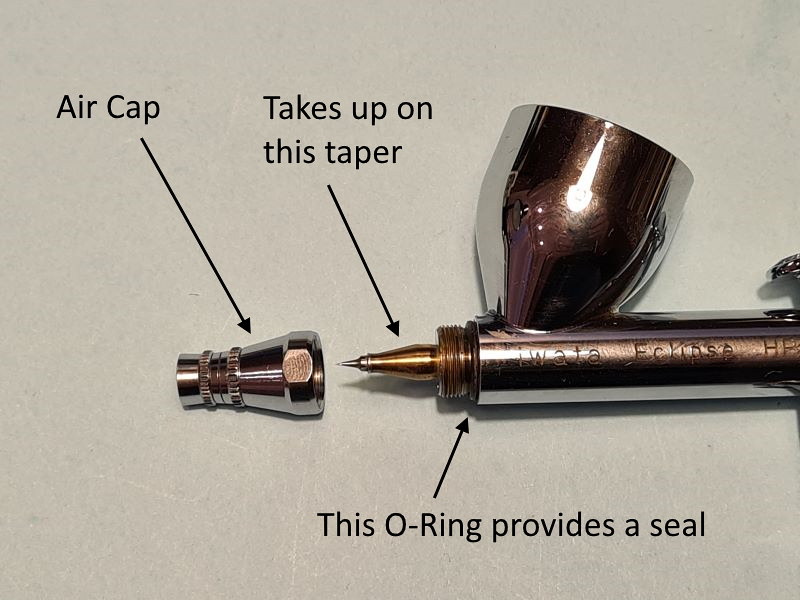The image portrays a detailed diagram of a sophisticated airbrush tool with a metallic copper finish, intricately labeled to identify each component. On the left sits a small metal air cap, which fits onto the taper of the primary nozzle section shown to the right. The airbrush features an O-ring that provides a seal just beyond the threads for secure attachment. Attached to the top of the nozzle is a large metal capture cup designed to hold various products for air spraying. The main body of the airbrush tool has faintly visible engraved text, seemingly reading "Iwata," against its silvery metallic surface. The entire assembly is shown against a neutral gray background, with arrows and text pointing to each part for clarity.